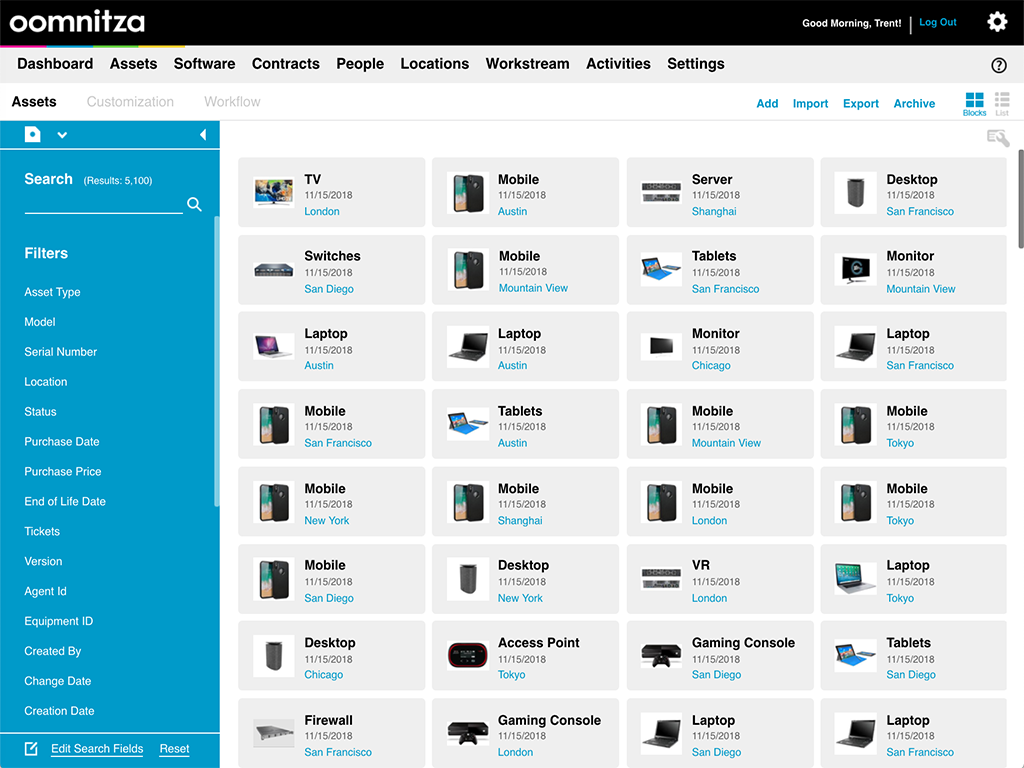This is a detailed screenshot of a website interface. At the very top, there is a black navigation bar with white text. On the left side, it reads "00MNITZA," while the right side warmly greets the user with "Good morning, Trent," followed by a vertical white line, a blue "Log out" link, and a small white gear icon for settings.

Below this top bar, a gray navigation menu spans the width of the page, displaying various options in black text from left to right: "Dashboard," "Assets," "Software," "Contracts," "People," "Locations," "Work Stream," "Activities," and "Settings." At the far right end of this bar, there is a small question mark icon enclosed in a circle, presumably for help or support.

Directly beneath the gray navigation bar, the page features a white rectangular section with the word "Assets" prominently displayed in black text. Accompanying this are "Customization" and "Workflow" links in gray text. Below these options, actions such as "Add," "Import," "Export," and "Archive" are highlighted in blue.

In the main content area, there are numerous gray squares arranged in a structured grid, likely representing individual items for sale or listing. The grid consists of eight rows, each containing four squares, making a total of 32 selectable items displayed neatly on the page.